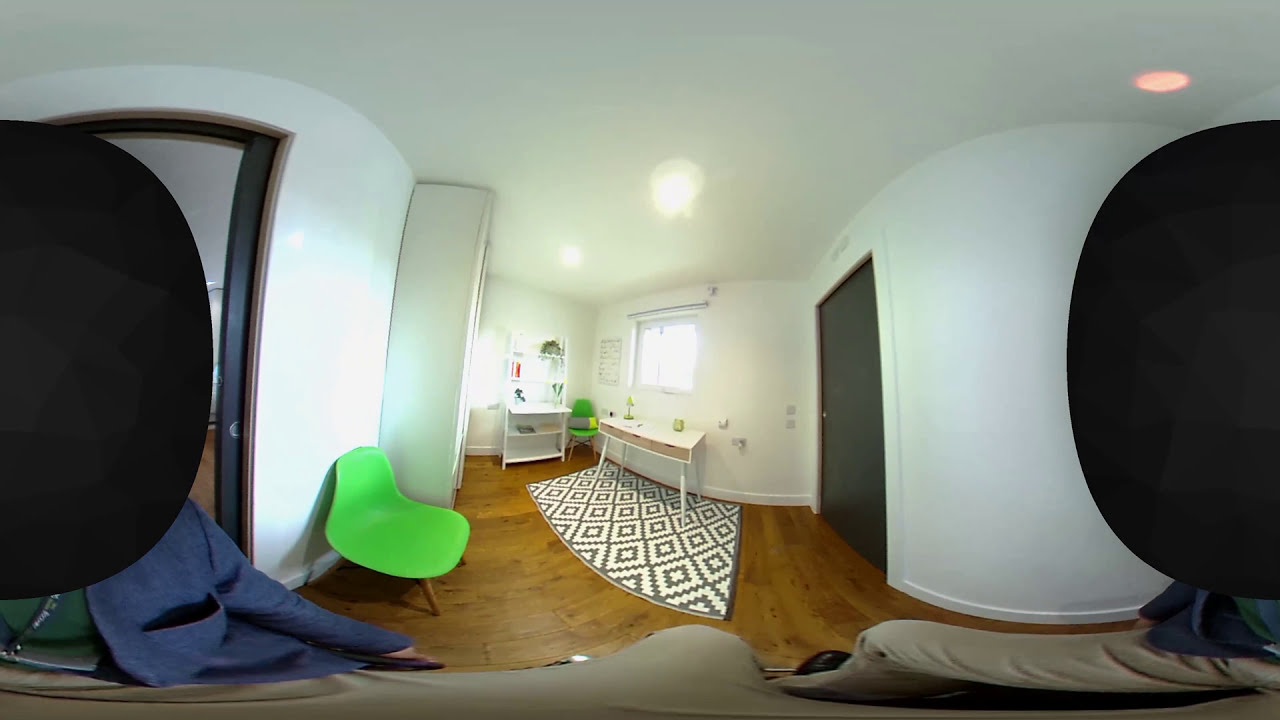This panoramic image captures a well-lit room with white walls and light brown hardwood floors. To the left, a black-framed door opens into a room with a notably warped, rounded wall. On the right, another black door remains closed, leading to another room with similarly rounded, white walls. Dominating the back of the room is a bright window with white light streaming through, directly above a white desk. This desk features a white top with brown shelves beneath and stands on four white legs, situated on a gray and white diamond-patterned rug. Adjacent to the desk, there is a white shelf touching the wall. In the lower-left side of the room, a plastic green chair, with light brown wooden legs, is placed against the wall near a large white wardrobe. In the upper right corner of the ceiling, an orange light dot is visible. The far left and right sides of the image are partially obscured by large black circular shapes, likely people’s heads, one revealing the torso of a person in a green shirt and blue jacket. The overall indoor setting suggests the photo was taken in the middle of the day, likely within an apartment.